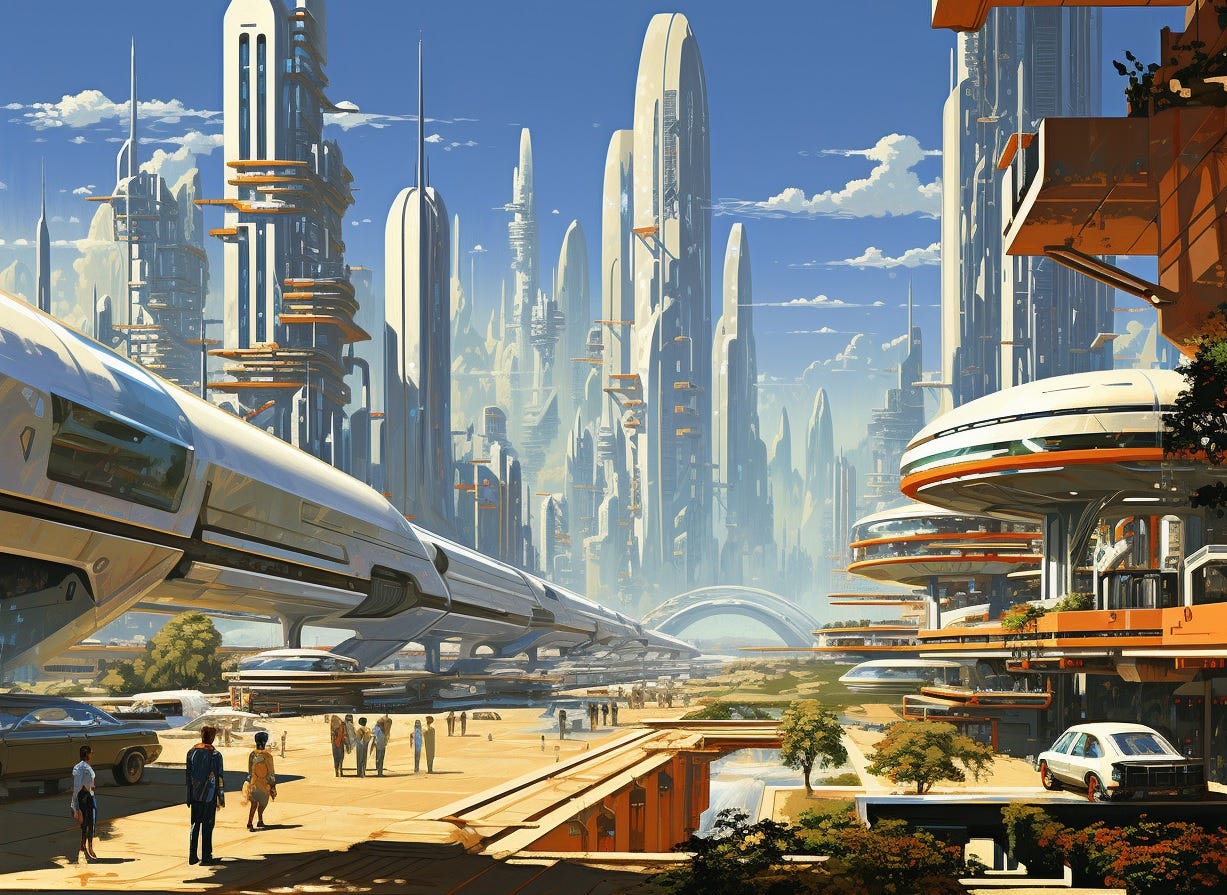The image is a meticulously detailed, futuristic cityscape rendered in a serious, cartoon-like style. From our vantage point on a street looking toward the city, we see numerous towering skyscrapers with a distinct rounded, rocket-like appearance and minimal visible windows. These buildings stand tall, evoking a sense of an advanced, almost alien civilization. On the street, primarily to the left side of the image, numerous people are walking away from the viewer, filling the boulevard with life.

Closer to us on the left, some smaller, rounded structures appear to serve as restaurants or offices, featuring curved windows that invite people to sit by their edges. Among these skyscrapers and rounded buildings, a current, ordinary-looking automobile stands out incongruously in the lower right corner, grounding the scene in the present despite its futuristic setting. Additional elements include sporadic trees amidst the predominately paved landscape.

A blue sky with scattered clouds stretches above the city, enhancing the contrast between the futuristic architecture and the familiar natural elements. In the distance, a track—perhaps for hyper-speed transit or a bullet train system—adds to the image's advanced technological feel. This depiction of an advanced, possibly dystopian city, blends elements of the fantastic with the ordinary, creating a vision of the future that feels both alien and eerily grounded in reality.